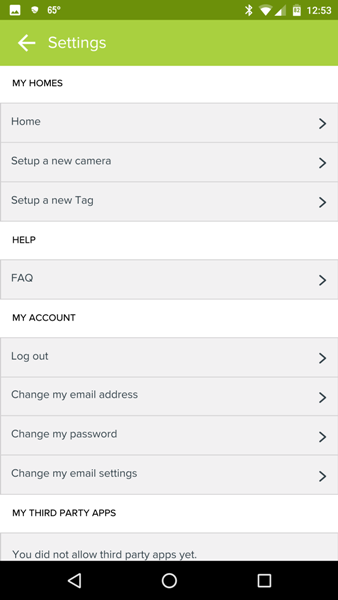The image displays a webpage interface, likely a settings page for a smart home management system. The top of the page features a green header that includes standard webpage informational icons and text. The main heading underneath this top section reads "Settings" with a right-facing arrow beside it, indicating a sub-menu.

Below this, there is a secondary heading titled "My Homes." Under this section, there are various clickable options, each accompanied by a right-facing arrow, including:
- "Home"
- "Set up a new camera"
- "Set up a new tag"

Following the home-related options, there is a "Help" section featuring another clickable entry labeled "FAQ."

Further down, a "My Account" section is listed, with several account management options, each with clickable arrows:
- "Logout"
- "Change my email address"
- "Change my password"
- "Change my email settings"

The final section on the page is "My Third Party Apps," which includes a message just above the bottom navigation bar indicating, "You haven't allowed third-party apps yet," suggesting that the individual is in the process of setting up or managing their system.